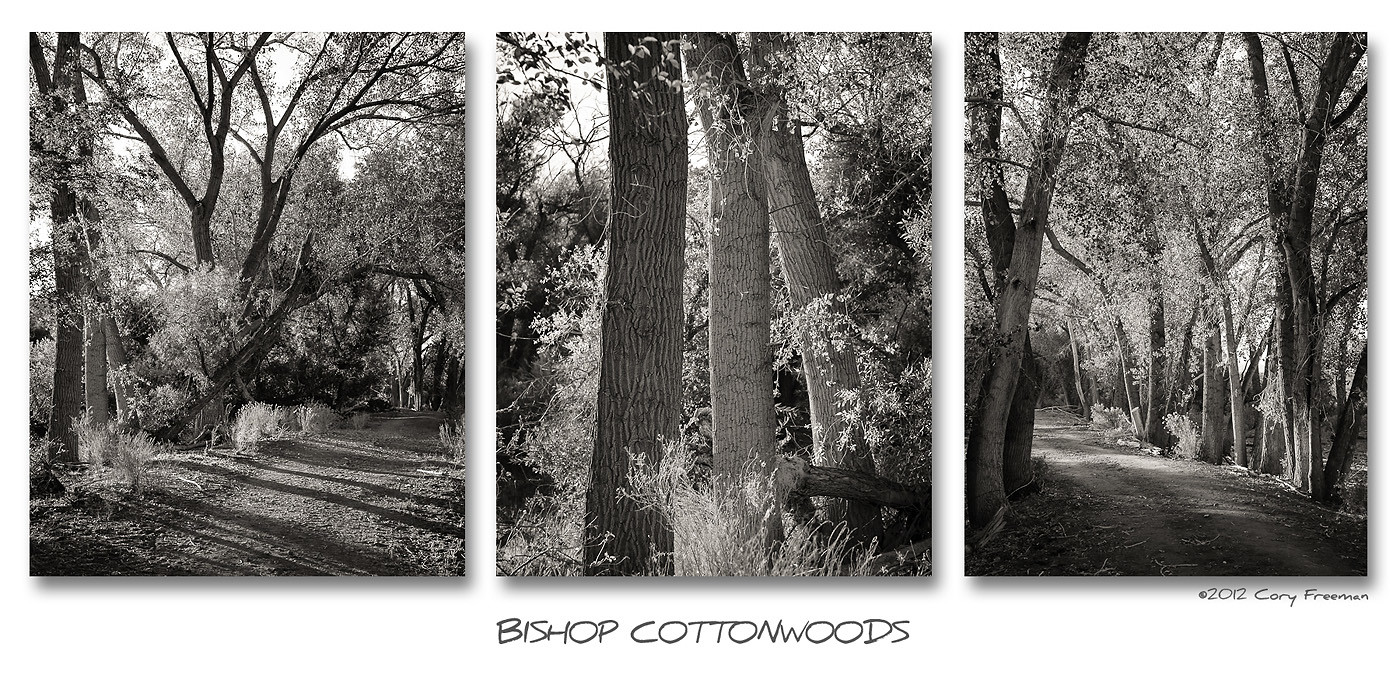The image is a set of three artistic photographs with a monochromatic palette, giving it a sepia-toned or gray-and-white appearance. Each of the three photos depicts various views of woodland scenes, featuring tall and seemingly blooming trees, suggesting a springtime setting. The photos are arranged side by side, appearing either mounted on a wall or given a slight shadow effect to create a three-dimensional look. The left and right images show towering trees flanking dirt pathways or roads, while the central photo is a close-up of three large tree trunks with no visible road. Beneath the trio of images, the text reads "Bishop Cottonwoods," and in the lower right corner, the photos are credited with "Copyright 2012 Corey Freeman."